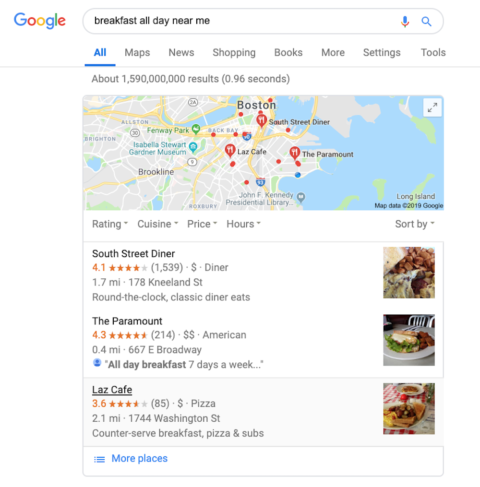This image is a screenshot taken from a Google Chrome browser, displaying the results of a search query for “breakfast all day near me.” In the top left corner, the Google logo is visible, followed by a search bar containing the query text. Below the search bar, a navigation menu lists options such as All, Maps, News, Shopping, Books, More, Settings, and Tools, with "All" highlighted in blue, indicating it is the active tab. 

The search results reveal approximately 1,590,000,000 results in 0.96 seconds. Beneath this information, a map of the Greater Boston area is displayed, marked with fork and knife icons indicating various restaurant locations. The map also shows bodies of water near Boston.

Below the map, the interface presents sortable categories including rating, cuisine, price, and hours. Featured establishments include South Street Diner, The Paramount, and Laz Cafe, each accompanied by a thumbnail image of the respective restaurant’s food. A link labeled "More places" is visible at the bottom, suggesting additional search results are available.